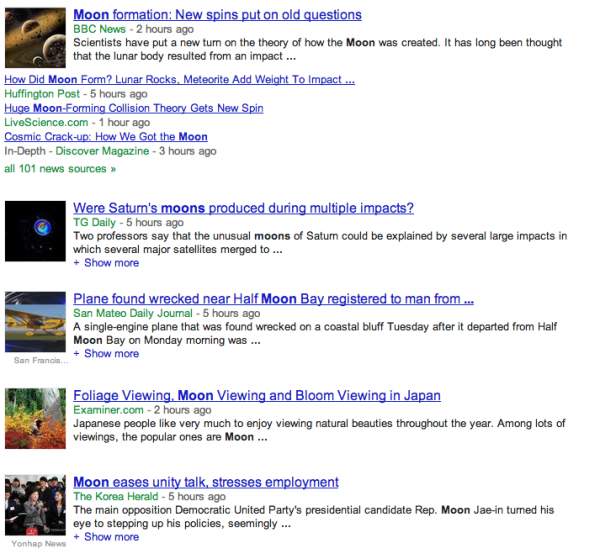The news webpage features a prominent section dedicated to recent scientific discoveries and events. At the top left corner, there is an image depicting outer space. Accompanying the image is a headline that reads: "Moon Formation: New Spins Put on Old Questions – BBC News, two hours ago." This article discusses the latest scientific perspectives on the formation of the moon, traditionally thought to result from a massive impact.

Additional headlines related to this topic include:
- "How Did the Moon Form? Lunar Rocks, Meteorite Add Weight to Impact" – Huffington Post, five hours ago.
- "Huge Moon-Forming Collision Theory Gets New Spin" – LiveScience.com, one hour ago.
- "Cosmic Crack-Up: How We Got the Moon" in-depth feature by Discover Magazine, three hours ago.

A link beneath these headlines reads: "All 101 news sources."

Further down the page, a second image of outer space, predominantly featuring a black background, accompanies another scientific inquiry: "Were Saturn's Moons Produced During Multiple Impacts?" – TG Daily, five hours ago. This article details theories by two professors suggesting Saturn’s unusual moons could be the result of several large impacts that caused major satellites to merge.

Another news icon features an airplane, accompanied by the headline: "Plane Found Wrecked Near Half Moon Bay, Registered to Man From…"

Below this, a thumbnail picture of foliage is associated with the topic: "Foliage Viewing, Moon Viewing, and Bloom Viewing in Japan."

The final thumbnail shows a group of people standing, with the headline: "Moon Eases Unity Talks, Stresses Employment" – The Korea Herald, five hours ago.